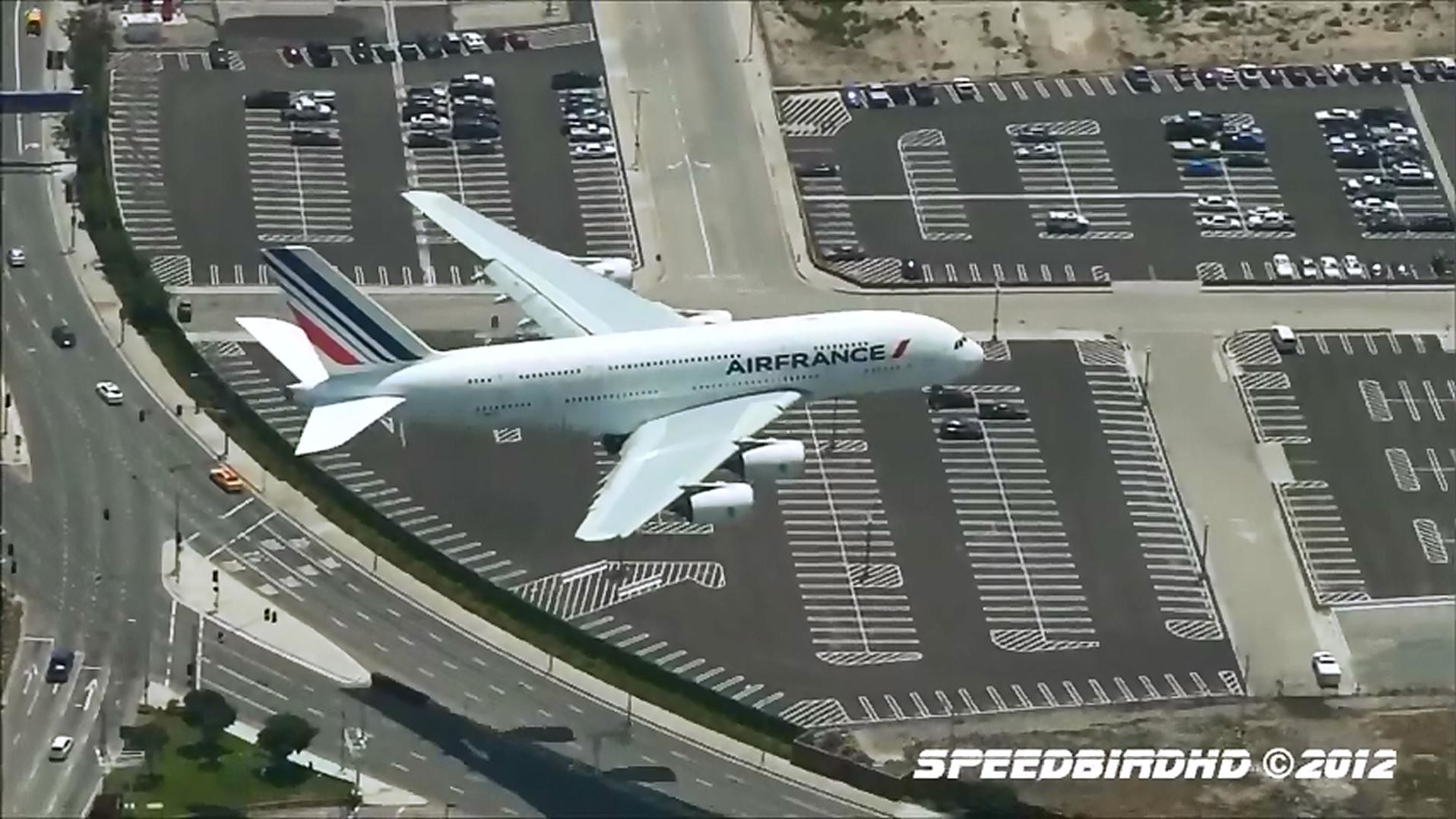A vivid photograph captures a silver Air France airplane flying low over a sprawling expanse of parking lots and multi-lane roads, possibly indicating proximity to an airport. The sun gleams brightly, casting a brilliant shine on the top of the aircraft. The parking lots, arranged in orderly sections, are mostly empty but do contain scattered parked cars. Adjacent to the parking area is a multi-lane highway with light traffic—just a few vehicles traversing the road. Surrounding the paved infrastructure, stretches of dry, desert-like terrain extend to either side, enhancing the sense of a remote airport environment. In the bottom right corner of the image, the text "Speedbird HD © 2012" is boldly displayed in white letters.